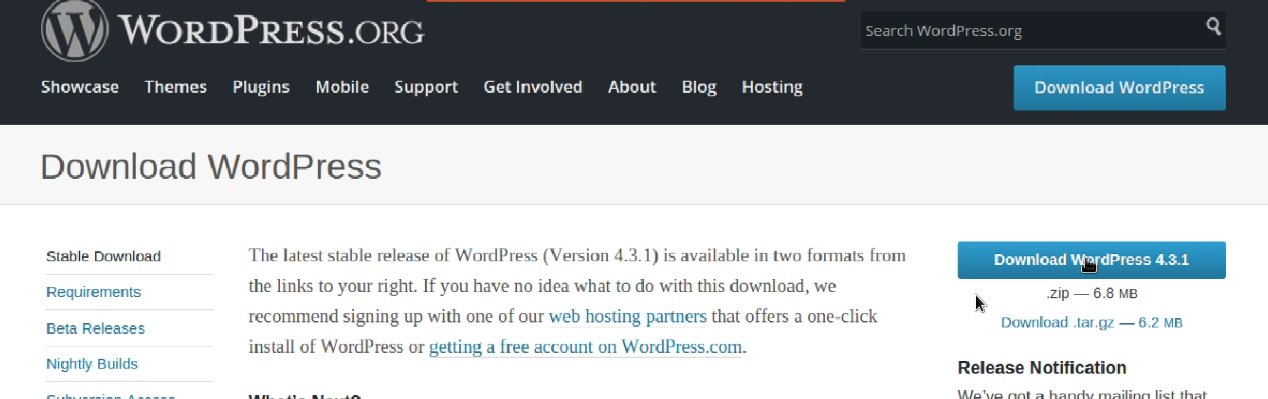The image is a screenshot from the WordPress.org website. At the top, against a black banner with white text, the WordPress.org logo is prominently displayed. The logo consists of a white "W" encased in a circle, positioned towards the left. On the far right of this banner, there is a search bar labeled "Search WordPress.org."

Below this banner, the background becomes white. At the top center, a blue button with white text reads, "Download WordPress." Directly below this, a horizontal navigation menu offers various clickable options: Showcase, Themes, Plugins, Mobile, Support, Get Involved, About, Blog, and Hosting.

Further down on the left side of the screen, there is a section titled "Stable Download" in black text. Below it, "Requirements" is listed in blue, followed by "Beta Release," "Nightly Builds," and another cut-off link, all in blue text.

On the right side of this section, descriptive text informs the user that the latest stable release of WordPress is version 4.3.1. It can be downloaded in two formats from the provided links. For users unfamiliar with the download process, it recommends signing up with a web hosting service. There is a blue "Download WordPress" link leading to a ZIP file, with an alternative format available underneath. A notification about the release is also present below these links.